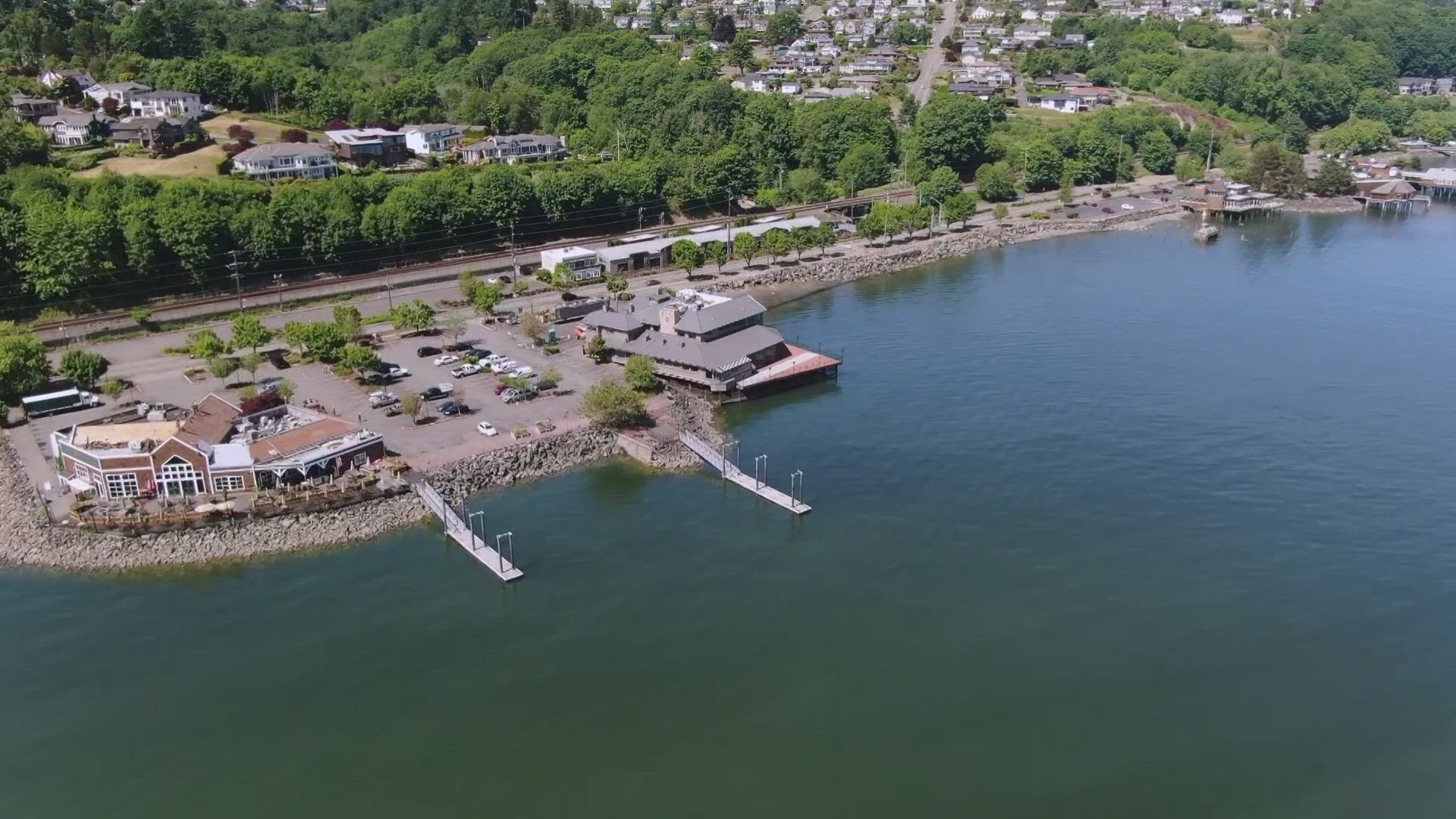This image is an aerial photograph of a picturesque waterfront landscape featuring a calm, green-watered bay. At the heart of the image, two substantial resort-style buildings flanking a sizable parking lot stand prominently. Extending from each building are docks that project into the serene waters, possibly serving as boat hangers. The shoreline is reinforced with a gray rock barricade, providing a sturdy boundary to the bay.

Adjacent to the shore and running parallel, there is a roadway accompanied by raised railroad tracks and power lines, delineating the separation between the waterfront and the residential area beyond. On one side of this division, towards the left, lie expansive, mansion-sized homes encircled by lush, mature trees and bushes, giving a sense of opulence and privacy. On the right side, in stark contrast, are smaller, more modest rambler-style homes.

Beyond the immediate coastal area, the scene includes a variety of houses nestled amongst thick tree lines, suggesting a verdant, possibly spring or summer setting with trees in full bloom. The entire scene is bathed in bright daylight, adding to the tranquil and inviting atmosphere of this picturesque landscape.